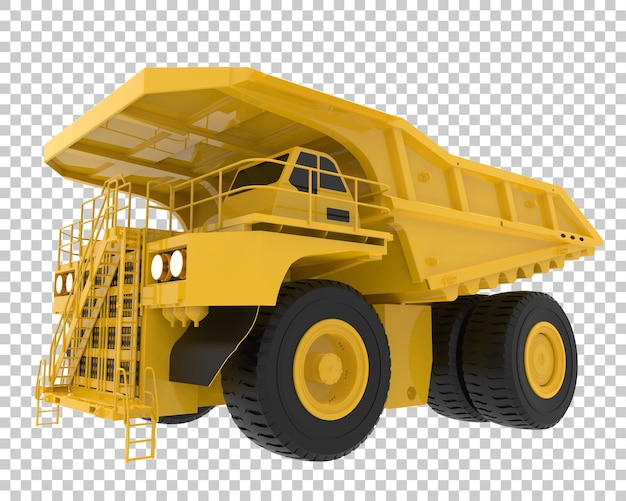The image is a highly detailed photograph of a miniature Tonka truck, prominently centered against a checkered background indicative of transparency. The truck resembles a heavy machinery vehicle often used in construction, fitted with a large loading or storage area at the top. Its eight enormous black rubber tires are fitted onto yellow rims, and the vehicle's imposing size necessitates the presence of ladders leading up to the driver's dark-tinted cabin. The truck, equipped with four glowing headlights, has a robust structure designed to handle and transport construction materials. This intricate toy model captures the essence of a real-life heavy-duty truck, complete with elaborate design elements such as a crane, multiple wheels, and functional components.